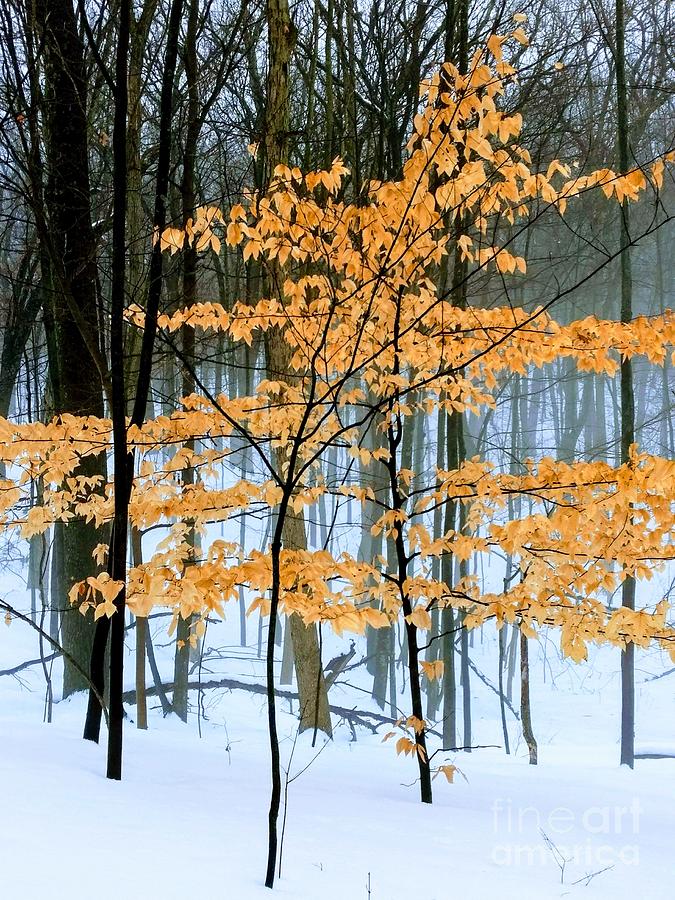This photograph captures a serene winter forest scene, with the ground blanketed in pristine, white snow. The focal point is a slender tree laden with vivid, bright orange leaves, standing front and center amidst an array of tall, bare trees that stretch their dark, leafless branches above the frame. The backdrop features a dense collection of these dead trees, their thin, twig-like trunks and branches creating a stark contrast against the snowy landscape. The sky, barely visible through the upper canopy, hints at a bluish-white, overcast day, adding to the chilly atmosphere. There is another similar tree with orange leaves peeking from the back right, further emphasizing the autumnal remnants clinging to the onset of winter. Some fallen branches are scattered on the snowy ground, and a slight haze in the background suggests rising vapor, possibly from the snow. The overall scene is devoid of people or animals, evoking a sense of peaceful solitude in this vividly beautiful winter forest setting. The bottom right corner of the photo includes the watermark "Fine Art America," indicating its artistic presentation.